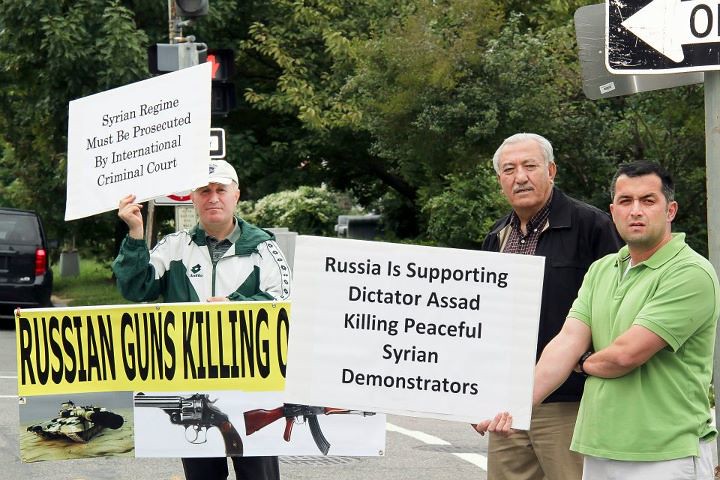The image depicts three aged male protesters standing at a street corner, each holding a sign critical of Russia's involvement with the Syrian regime. The signs read: "Syrian regime must be prosecuted by International Criminal Court," "Russian guns killing," and "Russia is supporting dictator Assad killing peaceful Syrian demonstrators." The protesters' attire includes a man in a green polo shirt with white shorts, another in a black jacket with a dark check shirt and khaki pants, and a third in a green and white windbreaker with a green shirt underneath, a white baseball cap, and dark pants. They are positioned near a metal pole with a partially visible one-way sign, and the scene is framed by abundant vegetation and trees lining the street. In the background, a car is parked on the street, emphasizing the residential nature of the area. There are also superimposed images of guns on the signs, underscoring the protest's message.